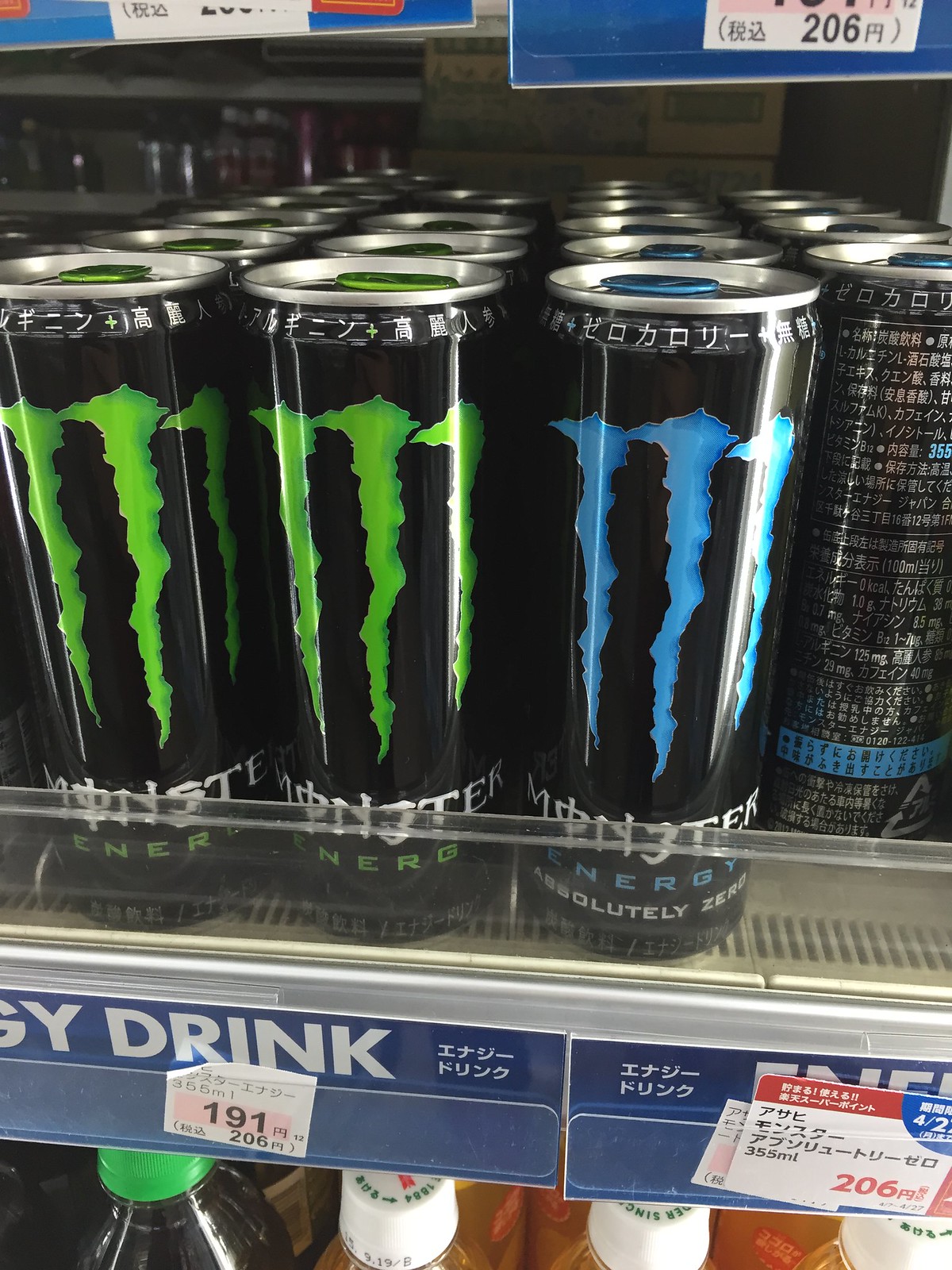This image captures a close-up view of a refrigerated shelf within a Japanese convenience or grocery store. The primary focus is on four columns of Monster Energy drinks, taking center stage in the middle of the frame. The majority of these cans are the standard black ones with the neon green "M" logo and "Monster Energy" text. Notably, one column on the right has a can missing, and another can in the same column is turned backward, revealing a blue "Zero Calorie" Monster Energy drink.

A plastic border runs across the shelf, and a blue and white banner at the bottom displays the words "Energy Drink" along with the pricing in Japanese text. Above the Monster cans, blue tags hang from the shelf. The shelf below is partially visible, showing the tops of various plastic bottle caps in different colors—green, white, and possibly other hues—highlighting the variety of drinks available in the refrigerated section. The entire setting is indoors, signified further by the cool, refrigerated backdrop.